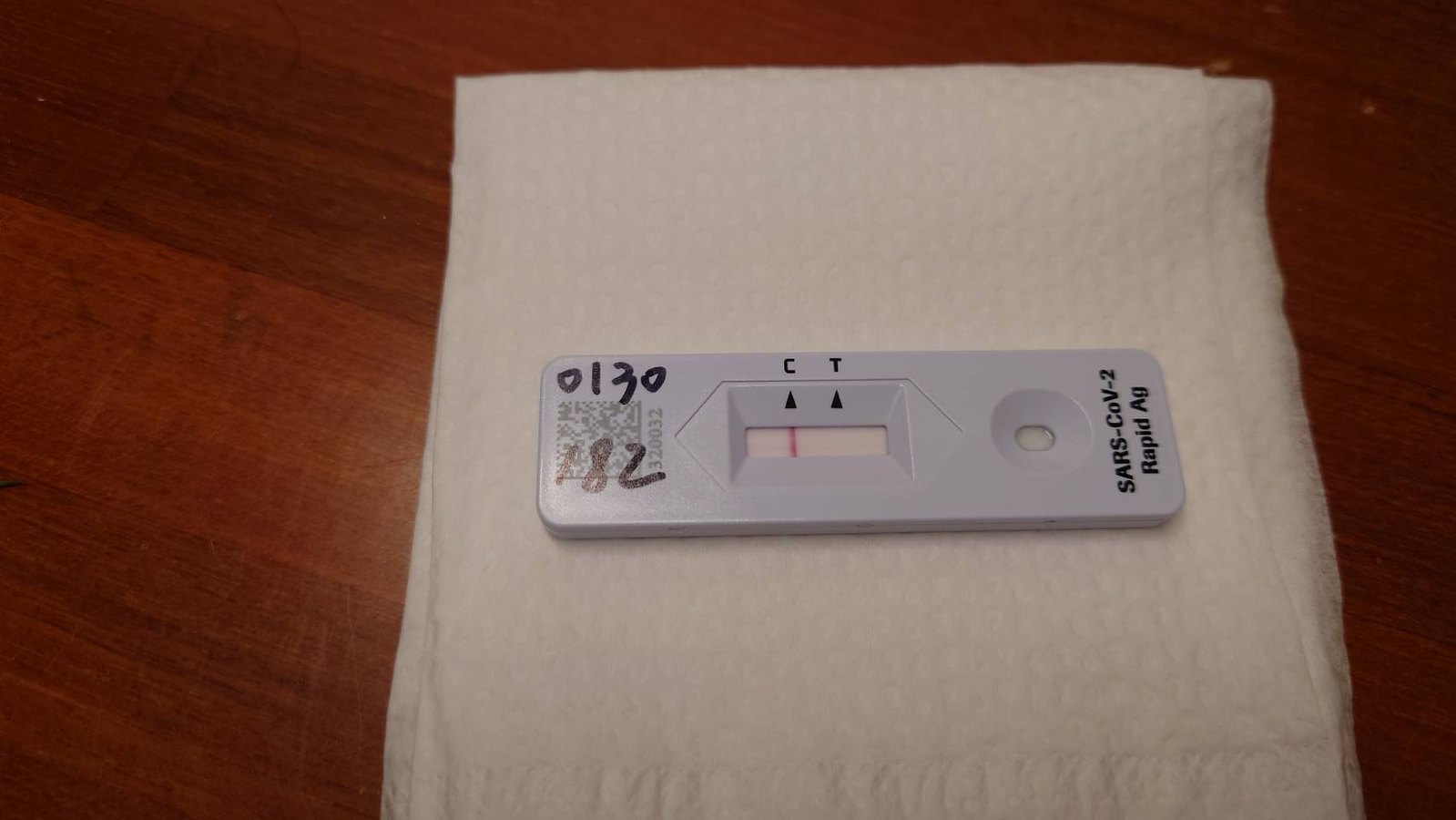This photograph captures a carefully arranged scene presented in landscape orientation. The background features a dark brown wooden table with visible streaks that run diagonally from the top left to the bottom right corner, adding texture and depth to the image. 

Placed centrally, but slightly off towards the top, is a meticulously folded white scarf. The scarf exudes a sense of luxury, reminiscent of soft, delicate cashmere. The bottom center reveals tiny, ruffled edges that accentuate its fine craftsmanship. The scarf's material is airy and light, with subtle indentations that hint at its fluffy texture. The right edge of the scarf is particularly translucent, underscoring its delicate nature. 

Resting atop this luxurious fabric is a gray plastic COVID-19 test, oriented horizontally from left to right. On the top left corner of the test, handwritten in marker, the numbers "0130" and "182" are visible, although the "182" appears to be faint and fading. The middle section of the test includes markings—a "C" and "T" each above a black triangle. A red mark under the "C" indicates a positive test result. To the right of these markings, a small clear circle reveals the scarf underneath. The far right end of the test is labeled "SARS-COV-2," with "rapid AG" inscribed below.

Overall, the composition juxtaposes the soft, fluffy nature of the scarf against the stark, clinical presence of the COVID test, creating a striking visual narrative.